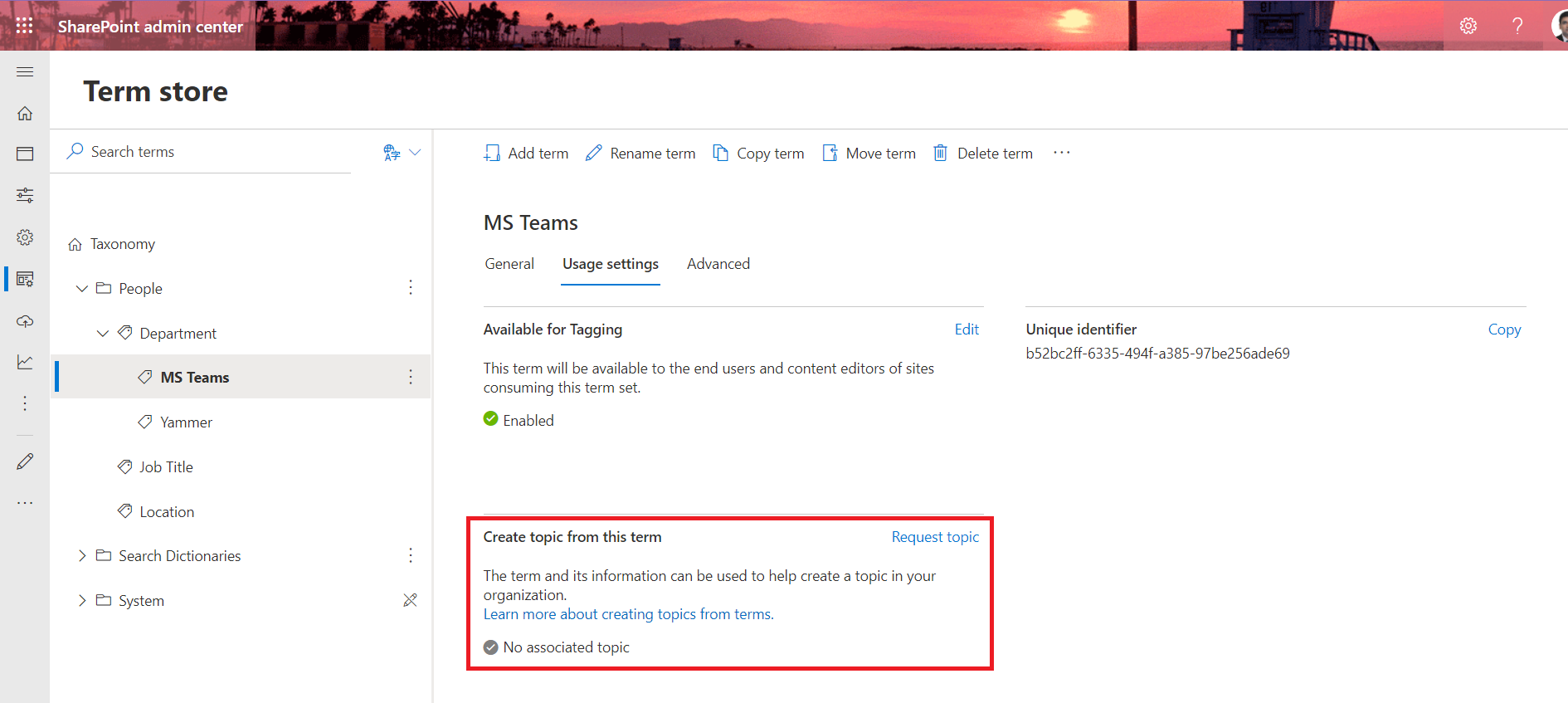A detailed, cleaned-up caption for the given image:

"A landscape-format, color screenshot captured from a laptop screen, showcasing the SharePoint Admin Center specifically within the Term Store section. The interface highlights a search area designed to locate specific terms. The available actions include adding, renaming, copying, moving, or deleting terms. The screenshot focuses on a term within the 'MS Terms' category, which is pertinent to Microsoft Teams, with an alternative choice being Yammer. A striking red rectangle emphasizes the 'Create Topic from this Term' option, underlined by a description that reads, 'The term and its information can be used to help create a topic in your organization. Learn more about creating topics from terms.' The interface further includes tabs like General, Usage Settings, and Advanced, providing comprehensive functionalities for term management within Microsoft Teams."